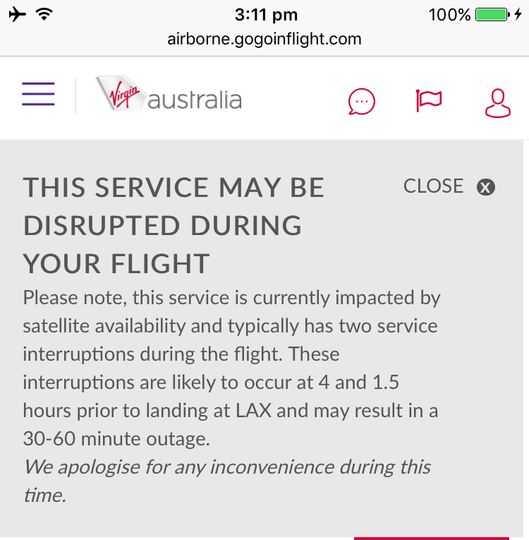The image is a screen capture from a mobile device, showcasing the user interface while the device is in use. 

The screen's background features a combination of white and light gray colors. In the upper left corner, the status bar displays the airplane mode icon, indicating that the device is currently in flight mode, along with the Wi-Fi signal icon. Centrally located in the status bar is the current time, showing as 3:11 p.m., with the URL "airborne.gogoinflight.com" positioned just below it.

On the upper right corner, the battery status is prominently displayed at 100%, accompanied by a green battery icon. 

Beneath the status bar, the visual is dominated by the logo of Virgin Australia—a red "Virgin" wordmark emblazoned on a distinctive white shape. This logo is prominently set against a light gray frame background.

Below the Virgin Australia logo, a light gray background contains an important notification in dark gray text. The advisory message reads: "This service may be disrupted during your flight. Please note, this service is currently impacted by satellite availability and typically has two service interruptions during the flight."

The overall image gives a clear and comprehensive view of the in-flight mobile interface, emphasizing the operational status icons, the time, and a service notice pertinent to the flight.